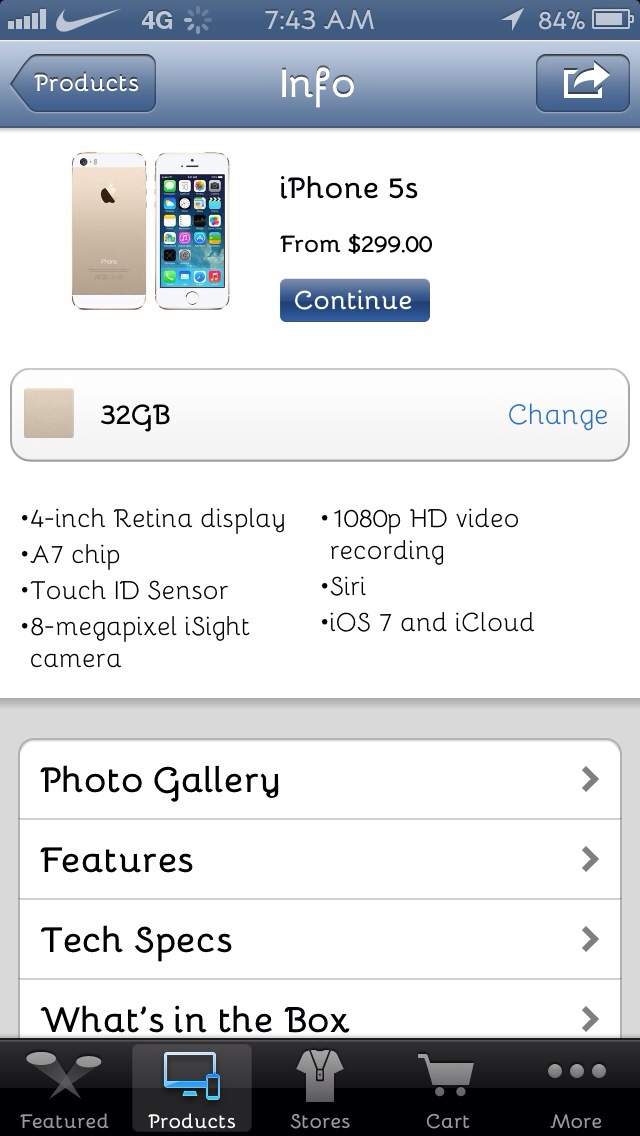The image is a detailed screenshot from a smartphone displaying a product page on a website. At the top of the screen, it indicates a 4G connection, the time as 7:43 AM, and a battery level of 84%. The header shows navigation buttons with a left arrow labeled 'Products' and 'Info' is centered, with a right arrow for exiting. Below this, the focal product is the iPhone 5S, listed at a starting price of $299. The device is specified to have 32GB of storage, highlighted by a blue 'Change' button. Key features of the iPhone 5S are detailed, including a 4-inch retina display, an A7 chip, a Touch ID sensor, an 8-megapixel iSight camera, 1080p HD video recording capabilities, Siri, iOS 7, and iCloud integration. Additionally, there is a blue 'Continue' button beneath the price. At the bottom, a menu provides options to view the photo gallery, features, tech specs, and contents of the box.